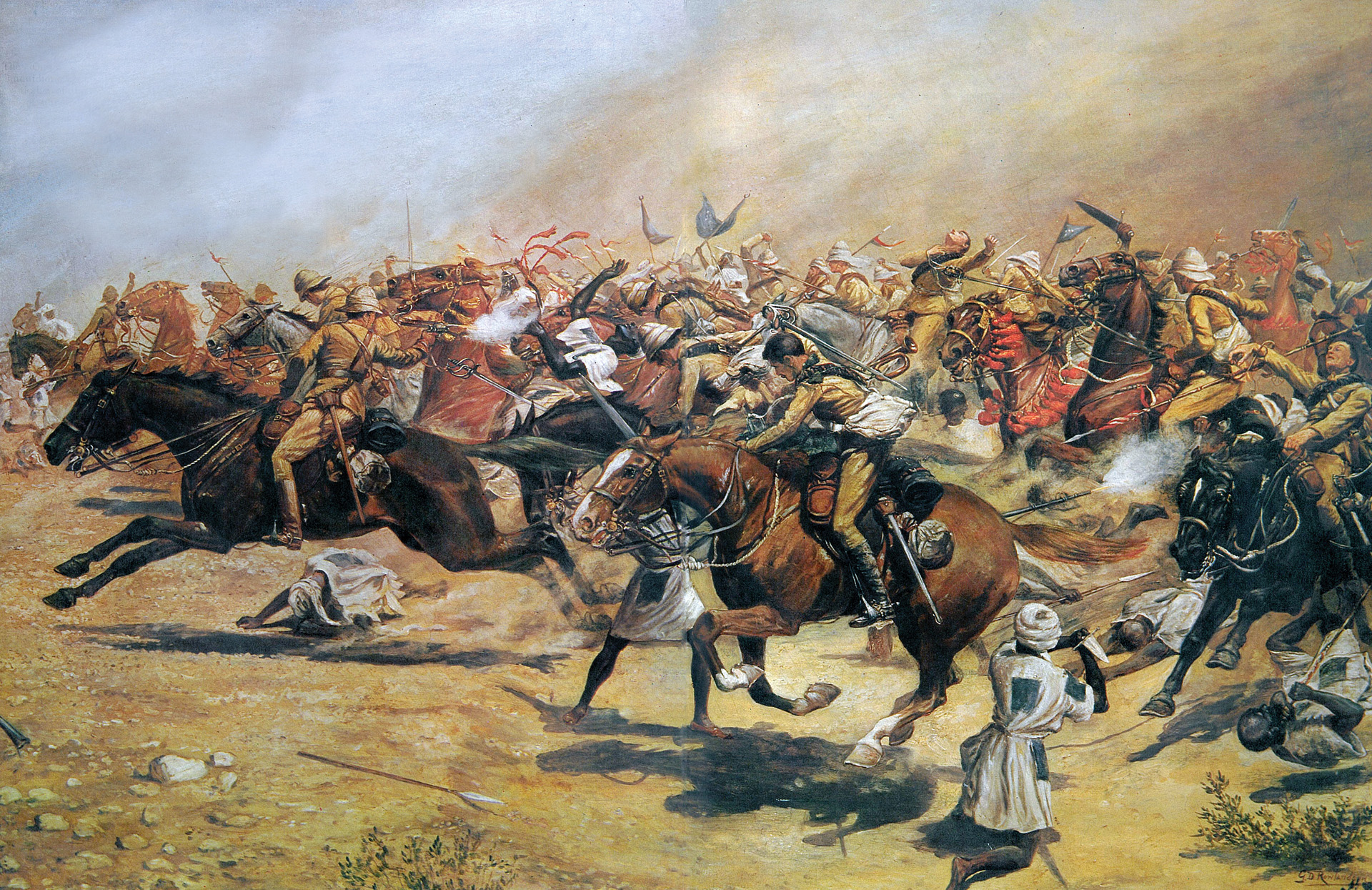This illustration captures a chaotic battlefield teeming with action and details. On the left side, numerous soldiers on horseback, predominantly in yellow uniforms with beige caps, wield gleaming swords and some firearms, emitting visible smoke. These men, some in metal helmets, surge forward, driving into the heart of the battlefield. Beneath them, clad in white garments with matching hats, are soldiers on foot, many of whom lay lifeless on the ground, pierced by weapons. The terrain is rocky and dusty, painted in shades of yellow and brown, with scattered bushes. In the smoke-filled sky, the tumult of battle is echoed by swirling clouds of dust. Amongst the turmoil, gray flags in the distance symbolize the ongoing conflict. The scene is a vivid depiction of the ferocity and chaos of war, underscored by the diverse colors of the horses and the smoky, indistinct background.